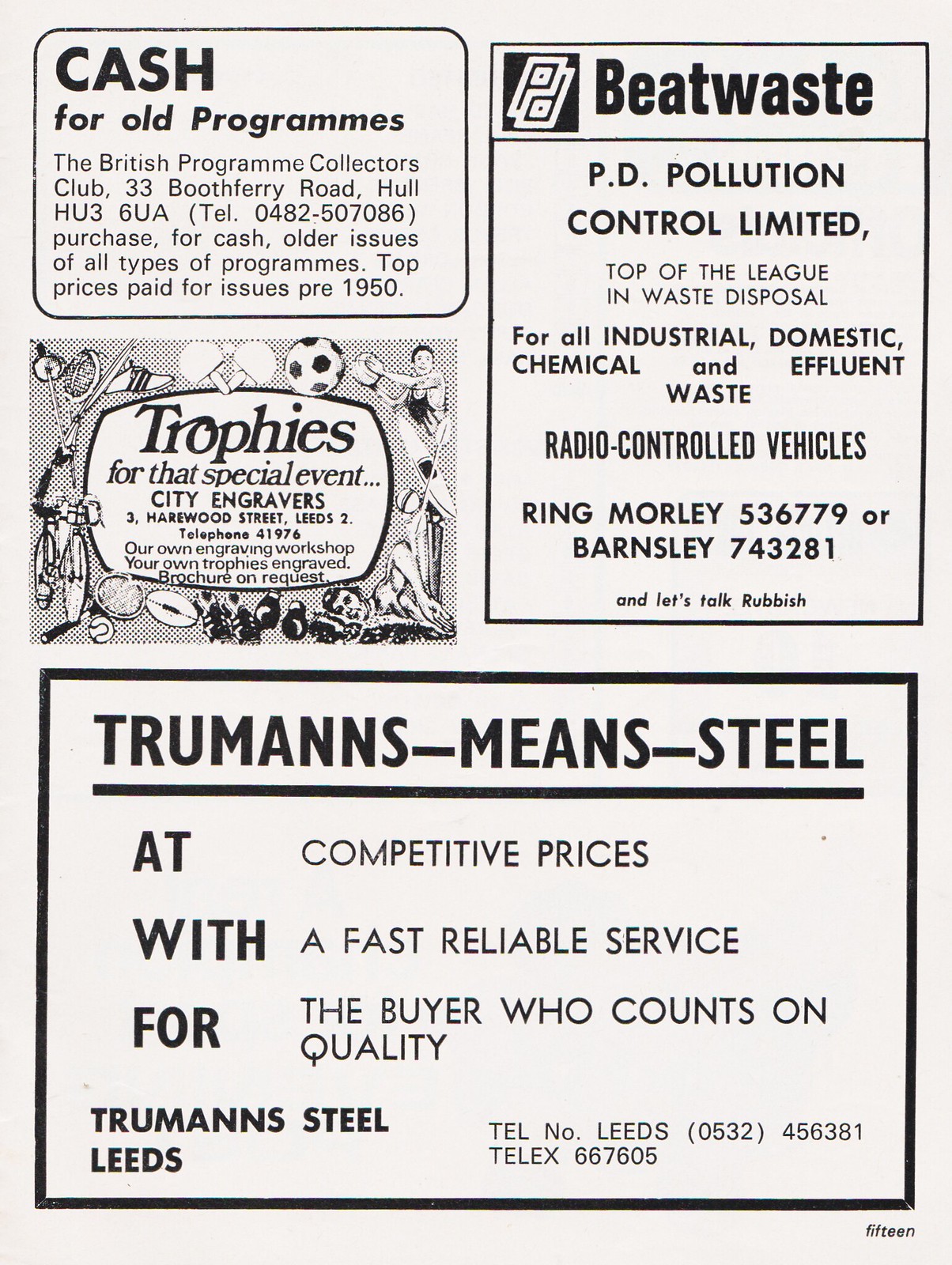The image is a black and white page from a sports event program filled with various advertisements. In the top left corner, there is an enclosed square that reads, "Cash for Old Programs, The British Program Collectors Club, 33 Booth Ferry Road, Hull HU3 6UA," and a telephone number, "040482-507086." Below this, surrounded by drawings of sports equipment, is an ad for "Trophies for Special Events by City Engravers," offering personalized engraving services and brochures upon request. On the right-hand side, another square advertises "Beat Waste, PD Pollution Control Limited, Top of the League in Waste Disposal," along with relevant contact numbers. Stretching across the entire bottom of the page is an ad for "Truman's Steel," highlighting "Competitive Prices with Fast, Reliable Service for the Buyer Who Counts on Quality," accompanied by phone numbers for further inquiries.